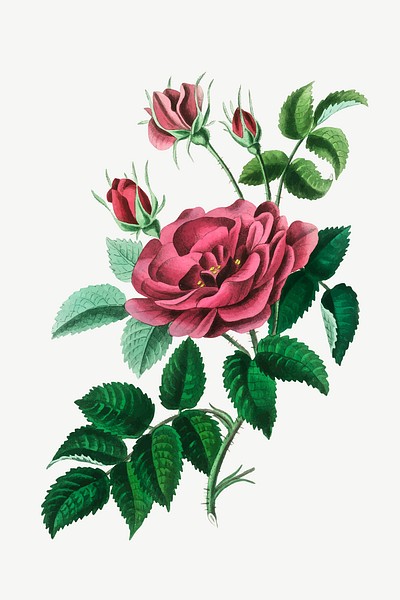This artwork is a detailed painting, likely done in acrylic, featuring a pink rose with a light blue background. The main focus is a lush, fully bloomed pink rose positioned centrally. Surrounding this prominent bloom are three additional rose buds at various stages of opening: one completely closed bud, another starting to open, and a third partially open. The plant features an intricate network of green stems and 18 pointed, dark green leaves, each with serrated edges. The leaves extend from the bottom of the painting toward the top and branch off in different directions, artfully filling the composition. The scene is cohesive, with the delicate details of the petals and foliage bringing the flower to life against the flat, light blue background.